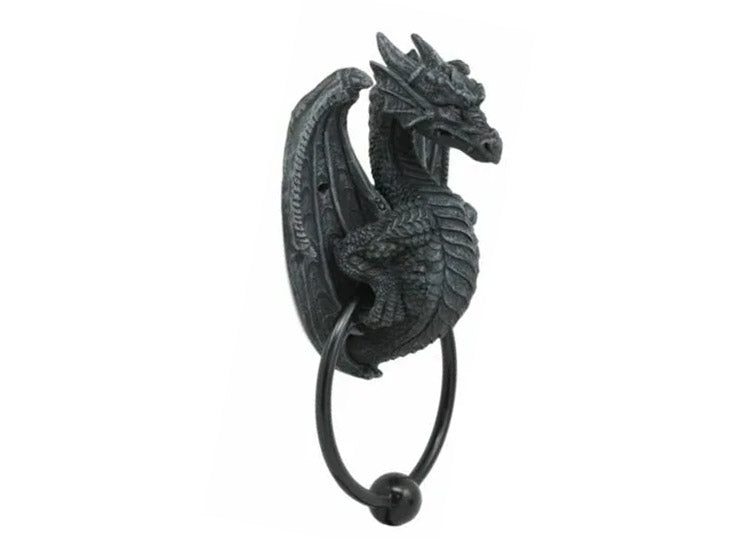The image depicts a detailed photograph of a dragon-shaped door knocker, centered against a stark white background. The dragon, rendered in shades of dark grey and charcoal, appears to be crafted from metal, exuding a gothic aesthetic. Its head, featuring prominent horns, points towards the right side of the frame. Bony, webbed wings extend behind it, curving from its back. From the middle part of its torso, a large, circular metal ring emerges, ending in a metallic ball at the bottom. This intricate design grants the functional hardware a mythical and formidable presence. The side-angled view of the door knocker allows for a clear display of its front and right-sided features, enhancing its three-dimensional appeal.